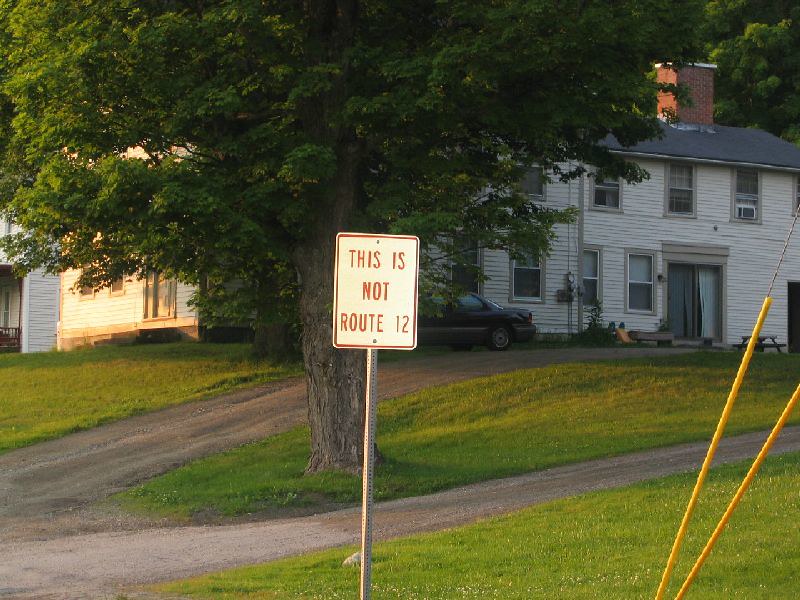The image depicts a slightly wider-than-tall scene, with the center featuring a distinct road sign mounted on a silver metal pole. The sign, ever so slightly tilted counterclockwise, is a white rectangle bordered in red and prominently reads "THIS IS NOT ROUTE 12" in red lettering. This sign appears before a residential setting, characterized by neatly trimmed grass and large trees slightly to the left of the scene. Behind the sign stands a substantial white house, which takes up the upper half of the image, flanked by an early 2000s sedan, indicating the era of the photo. To the right, two yellow lines—possibly road markings—are visible, though what they delineate remains unclear. The road extends out, suggestively leading into the residential area.